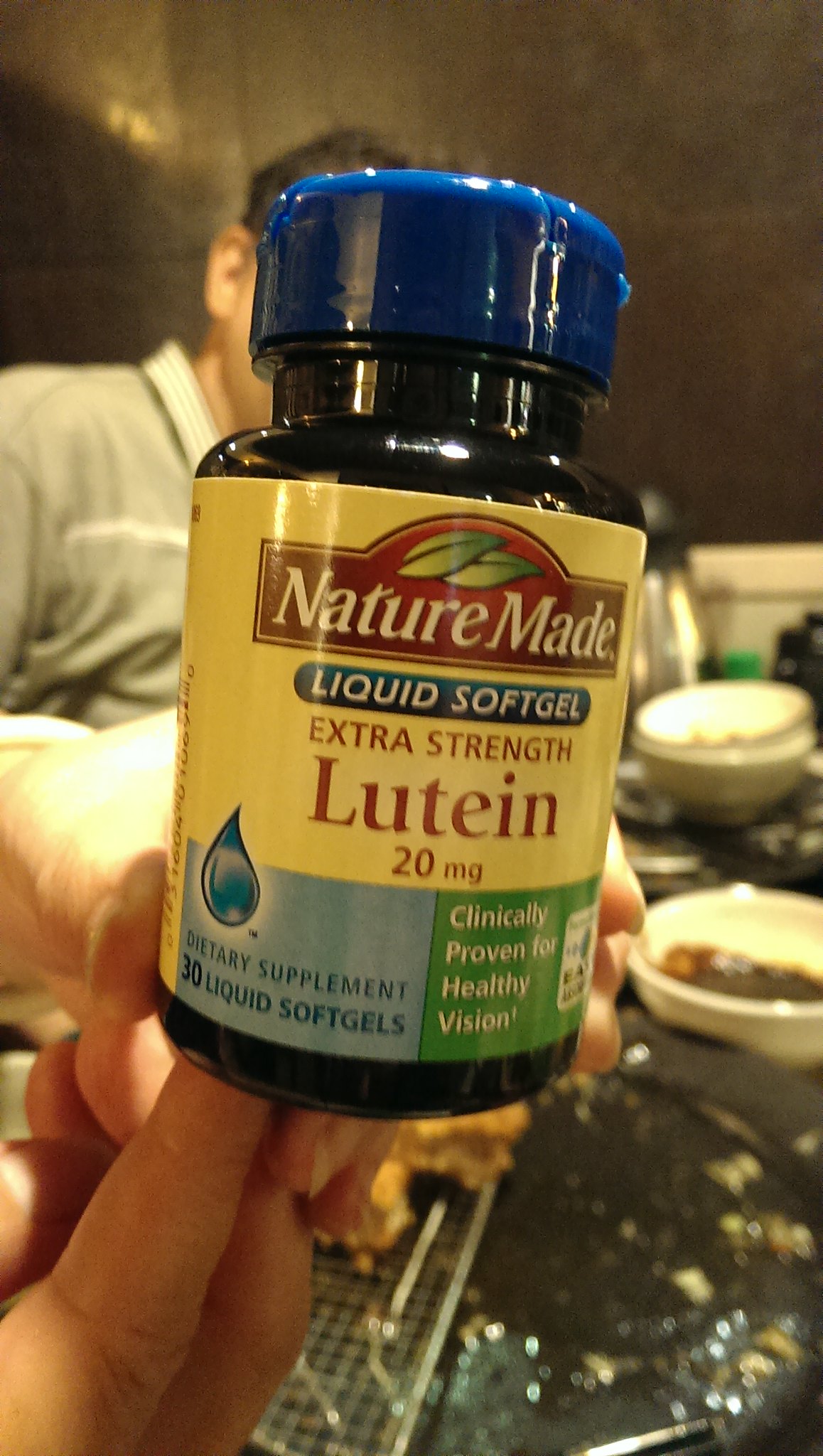In this vertical rectangular photograph, a person holds up a shiny, dark brown plastic bottle of vitamins with a translucent blue cap and a large yellow label. The label prominently features the text "Nature Made" in white letters outlined in red. Beneath that, in red text, it reads "Liquid Soft Gel Extra Strength Lutein 20 mg." On the lower part of the label, there are sections with blue and green backgrounds stating "Dietary Supplement, 30 Liquid Soft Gels" and "Clinically Proven for Healthy Vision" in blue and white text, respectively.

The setting appears to be indoors with a dark background, and visible on the table are a few bowls. Behind the bottle, another person, likely male with dark brown hair and wearing a white shirt, is partially visible. The light reflecting off the bottle creates a speckled, shiny appearance, highlighting its glossy surface.